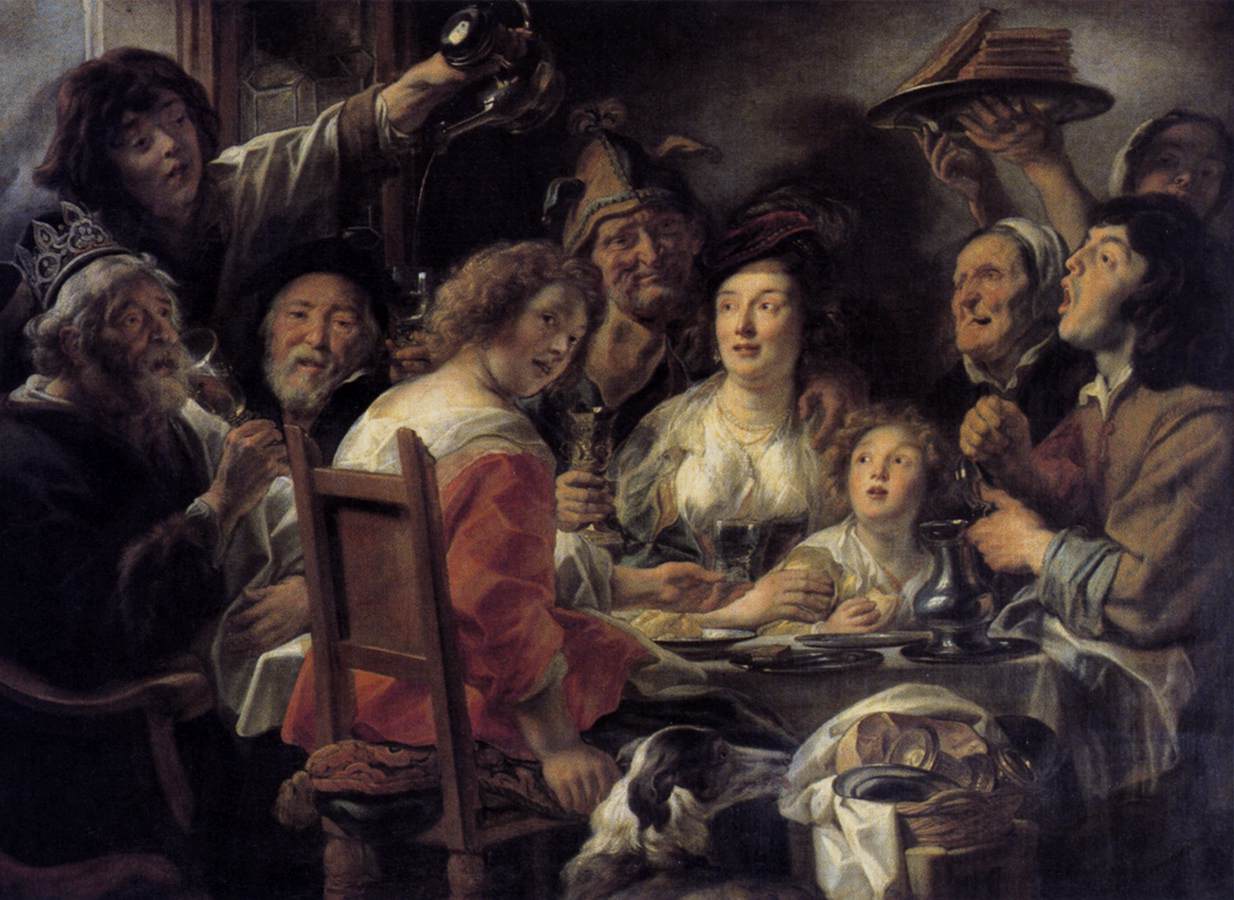The artwork, entitled *The King Drinks* by Jacob Jordaens, is a large square painting from the Renaissance period, predominantly featuring muted colors with touches of orange and red. Central to the scene, a woman in an orange-red dress with a white scarf and brown hem sits in a high-backed wooden chair, her body facing the table but her head turned toward the viewer with a surprised expression. Surrounding her, about ten people are gathered around a wooden table adorned with black dinner plates and bread. 

To her left sits an older man, notable for his crown and regal black attire with a white scarf, suggestive of his status as a king. He has white hair and a thick beard and mustache. Adjacent to him is a man wearing a black hat, and another with a unique cap that extends upwards with two points, possibly indicating armor. Across the table stands a woman holding a chalice, clad in a white outfit and hat, her upper body visible. 

A dynamic and lively atmosphere pervades the painting, with various figures caught in gestures of conversation, shouting, and laughter. In the background, another woman carries a tray laden with bread. A few characters are striking: an older man with a gray beard, a helmeted figure in the center back, an elderly woman in a white cap who appears toothless, and a young child eating bread.

On the right side of the painting, a black and white dog, possibly a greyhound or whippet, sits beside a basket of dirty dishes. The overall scene is set against a background of dark brown and black, enhancing the intimate and bustling ambiance of this indoor dining room gathering.